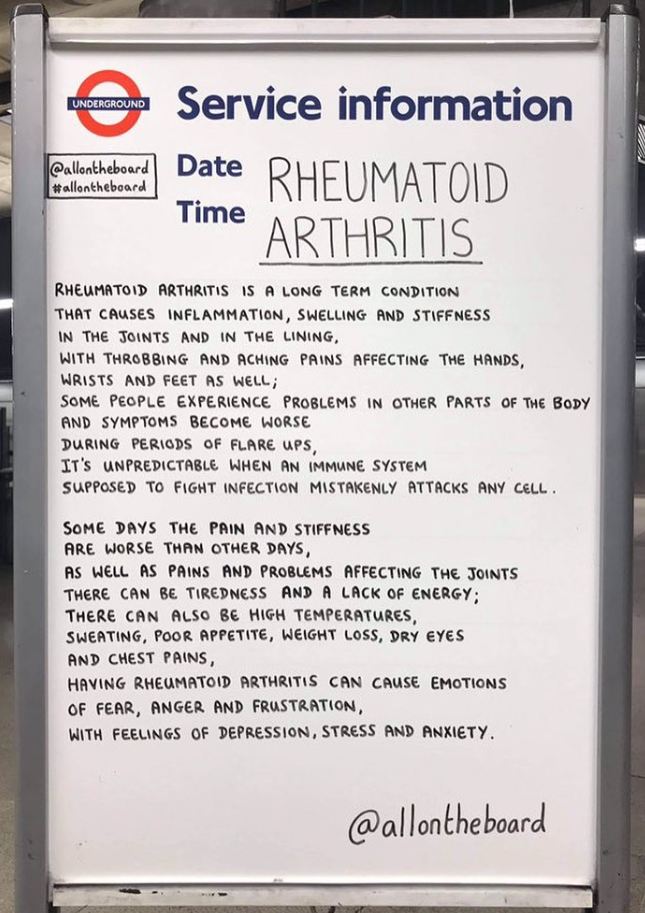The image is a color photograph in portrait orientation, focusing on a white informational poster set within a chrome-colored frame. The top left corner of the poster features a circular red logo with a dark blue horizontal banner across its center, bearing the white text "UNDERGROUND." To the right of this logo, in larger blue text, is the heading "SERVICE INFORMATION." Below this heading, in black handwriting, are the words "DATE" and "TIME," followed by "RHEUMATOID ARTHRITIS."

The main body of the poster provides detailed information about Rheumatoid Arthritis, a long-term condition causing inflammation, swelling, and stiffness in the joints, with symptoms including throbbing and aching pain affecting the hands, wrists, and feet. The text describes how some people may experience additional issues in other parts of the body, and it highlights the unpredictability of symptom flare-ups, which can vary in severity from day to day. Additional symptoms mentioned include tiredness, lack of energy, high temperatures, sweating, poor appetite, weight loss, dry eyes, and chest pains. The emotional impact of the condition is also noted, with references to feelings of fear, anger, frustration, depression, stress, and anxiety.

The bottom right section of the poster bears the handwritten text "At All on the Board," which is repeated at the top left of the poster next to the date information. For further information, viewers are directed to visit www.FEMA.gov. The overall style of the poster combines photographic representationalism and realism, emphasizing clear presentation and detailed information.